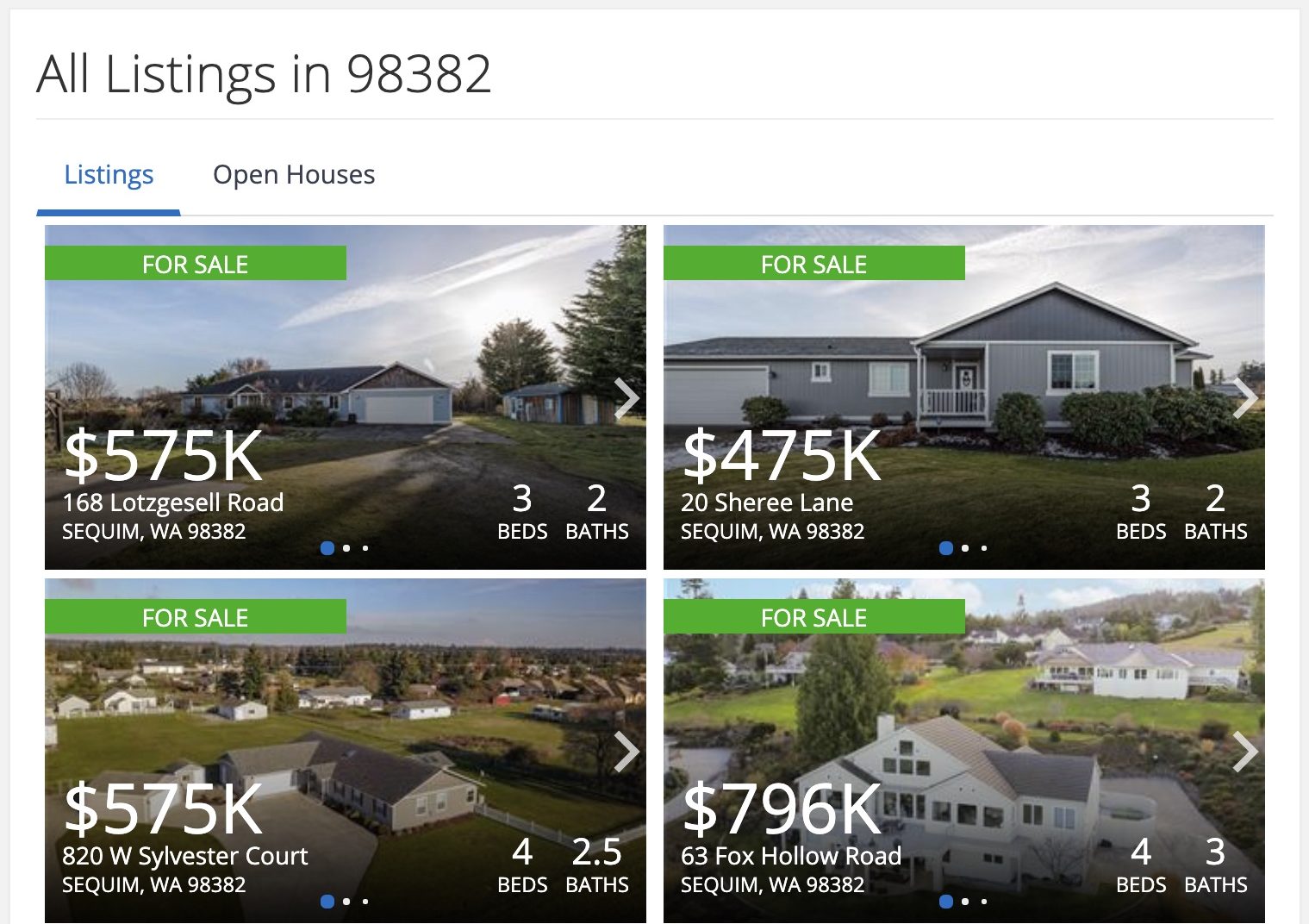A screenshot showcasing real estate listings in the 98382 zip code (Sequim, Washington). The interface features the heading "All Listings in 98382." At the bottom, there are tabs for "Listings" and "Open Houses." The visible listings include:

1. A house for sale at $575,000. It offers three bedrooms and two bathrooms.
2. Another home listed at $475,000, located on 20 Sherry Lane, with three bedrooms and two bathrooms.
3. A third property with four bedrooms and two and a half bathrooms, priced at $575,000. The image appears to be an aerial shot, possibly taken with a drone.
4. The fourth listing shows a house with four bedrooms and three bathrooms, priced at $796,000.

The arrows at the ends of the listings suggest that more listings are available but not visible in this particular image.